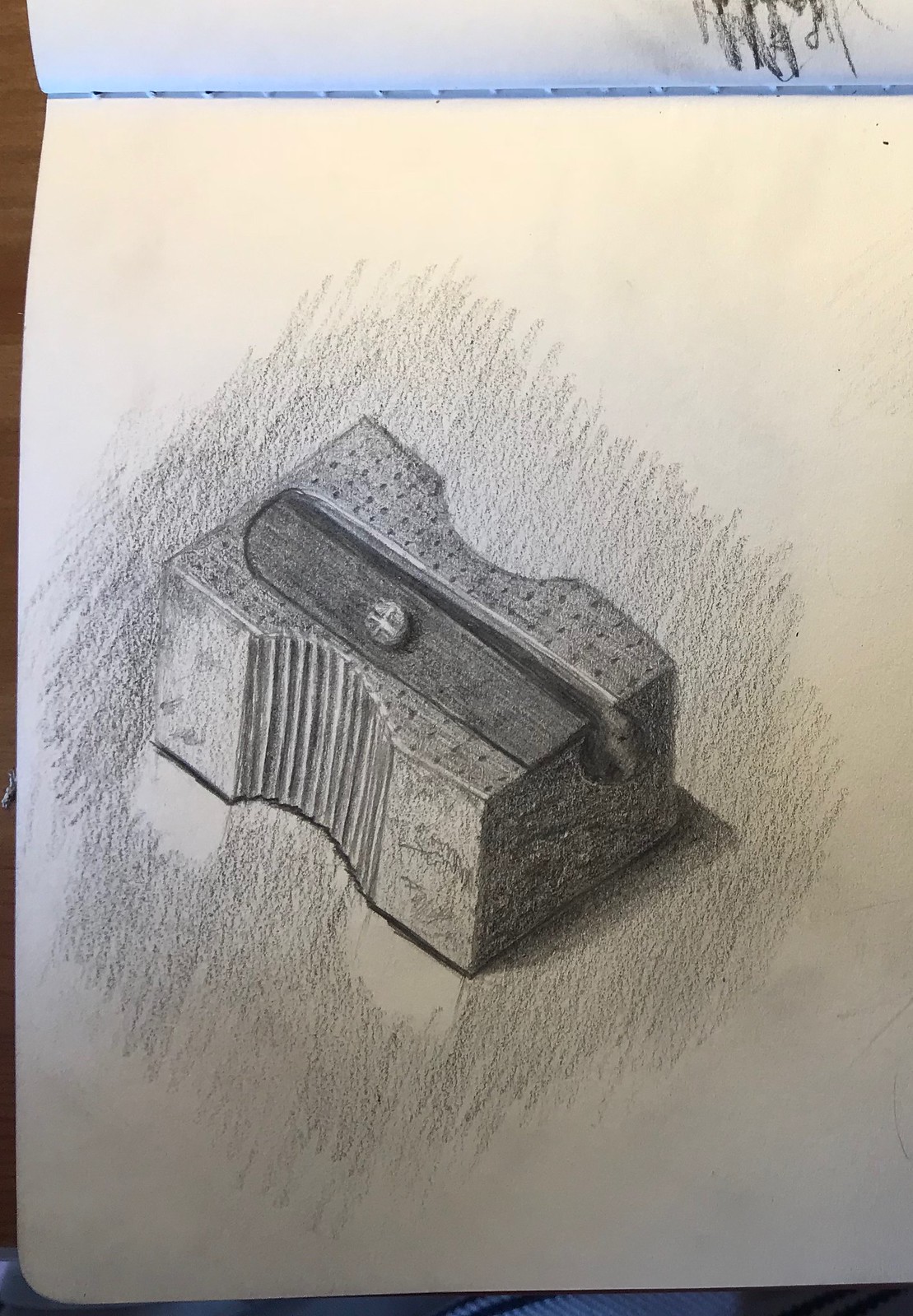This detailed pencil drawing, captured in a vertically aligned photograph, depicts a small, steel pencil sharpener. The sharpener features a small opening in the bottom right corner, just large enough to insert a wooden pencil for sharpening. The central part of the sharpener houses a blade, secured by a small screw, which shaves the pencil to a fine point when turned. The design includes two ergonomic grips on either side, making it easy to hold while sharpening. The artist has skillfully shaded the drawing to give it a three-dimensional effect, emphasizing the metallic texture of the sharpener. Surrounding the sharpener are several pencil shavings, enhancing the realism of the scene. The drawing is done on white paper, likely part of a sketchbook, as indicated by the folded-over paper at the top of the image. The entire scene is meticulously rendered in black and white, showcasing the artist's attention to detail.